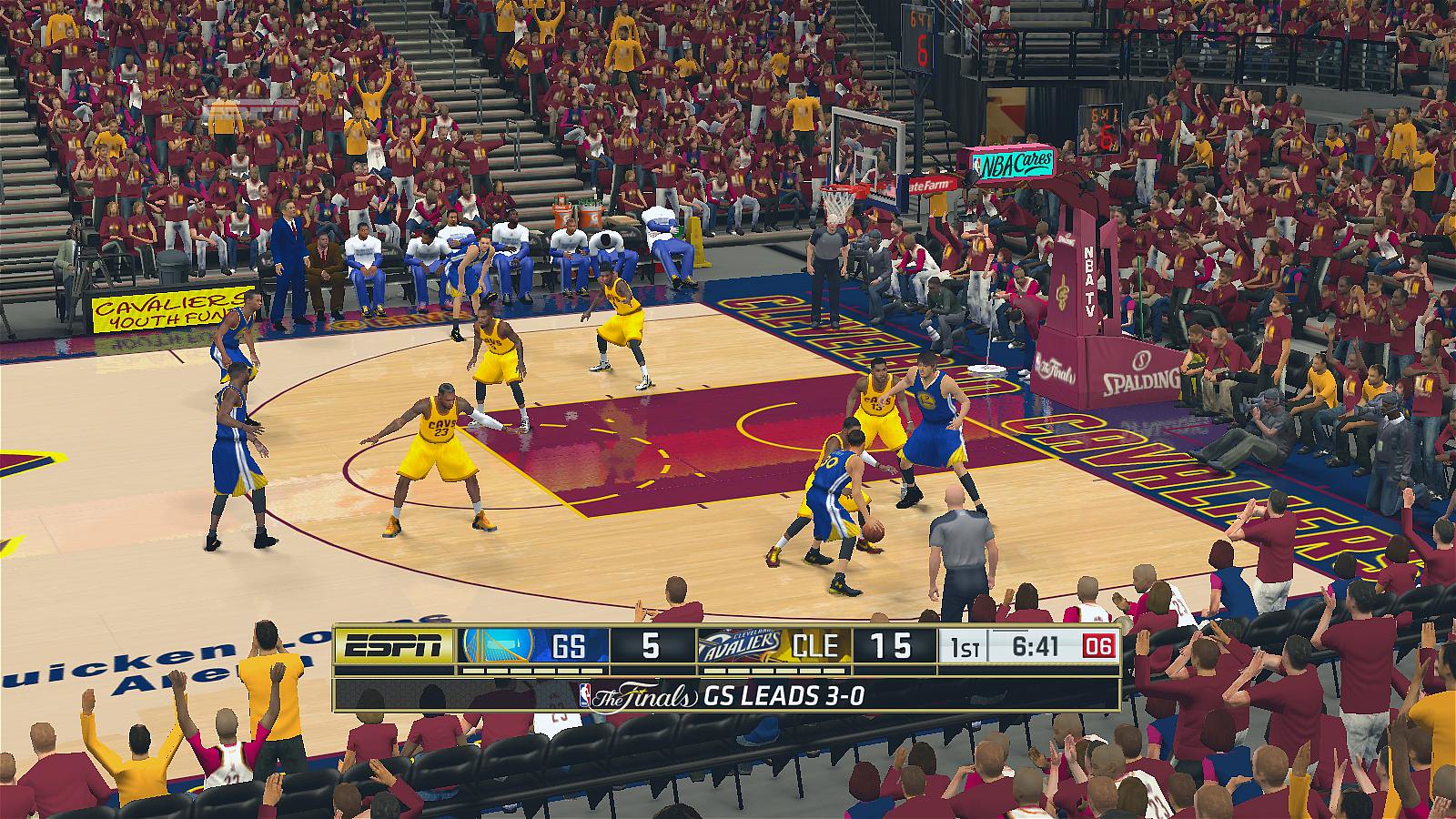The image is a screen capture from a basketball video game featuring a match between the Cleveland Cavaliers and a team likely to be the Golden State Warriors. The Cavaliers are playing at home, evident from the maroon and gold colors adorning the stadium floor, which reads "Cleveland Cavaliers". In the scene, players rendered with a plastic-y, computer graphics look add to the distinct video game aesthetic. The game action features players in yellow jerseys forming a defensive formation around their basket, while a player in a blue and white jersey holds the basketball, suggesting the Warriors are in possession.

A less detailed crowd surrounds the arena, with many fans dressed in Cleveland's maroon and gold colors, some with their hands in the air, showcasing their excitement and support. At the bottom of the image, a scoreboard strip displays the ESPN logo in black, followed by "GS5 CLE15" in white, indicating the Cavaliers lead 15-5. Additional text reads "FIRST 6:41," presenting the first quarter with six minutes and forty-one seconds remaining.